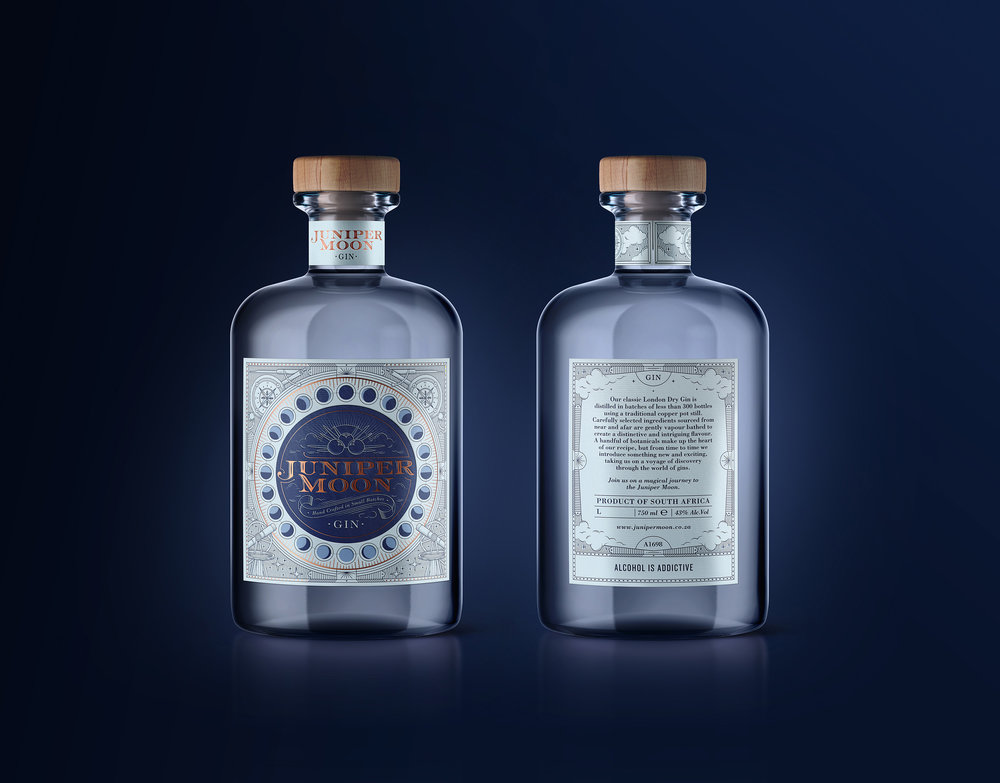The image features two bottles of Juniper Moon Gin against a dark blue background, with the center of the image highlighted in a lighter blue. The bottle on the left displays the front label prominently, showcasing the name "Juniper Moon Gin" in copper-colored text and a small neck label bearing the same name. Both bottles are capped with gold-toned, wooden lids. The bottle on the right reveals the back label, which contains a detailed description of the gin and its origin, stating it is a product of South Africa. The label also includes a silhouetted image of a landmark or continent in gray and white tones. At the bottom of the back label, there is a warning that alcohol is addictive. The gin bottle itself is made of blue glass, and the image is backlit to emphasize the bottles' shapes, creating a minimalistic and elegant design.